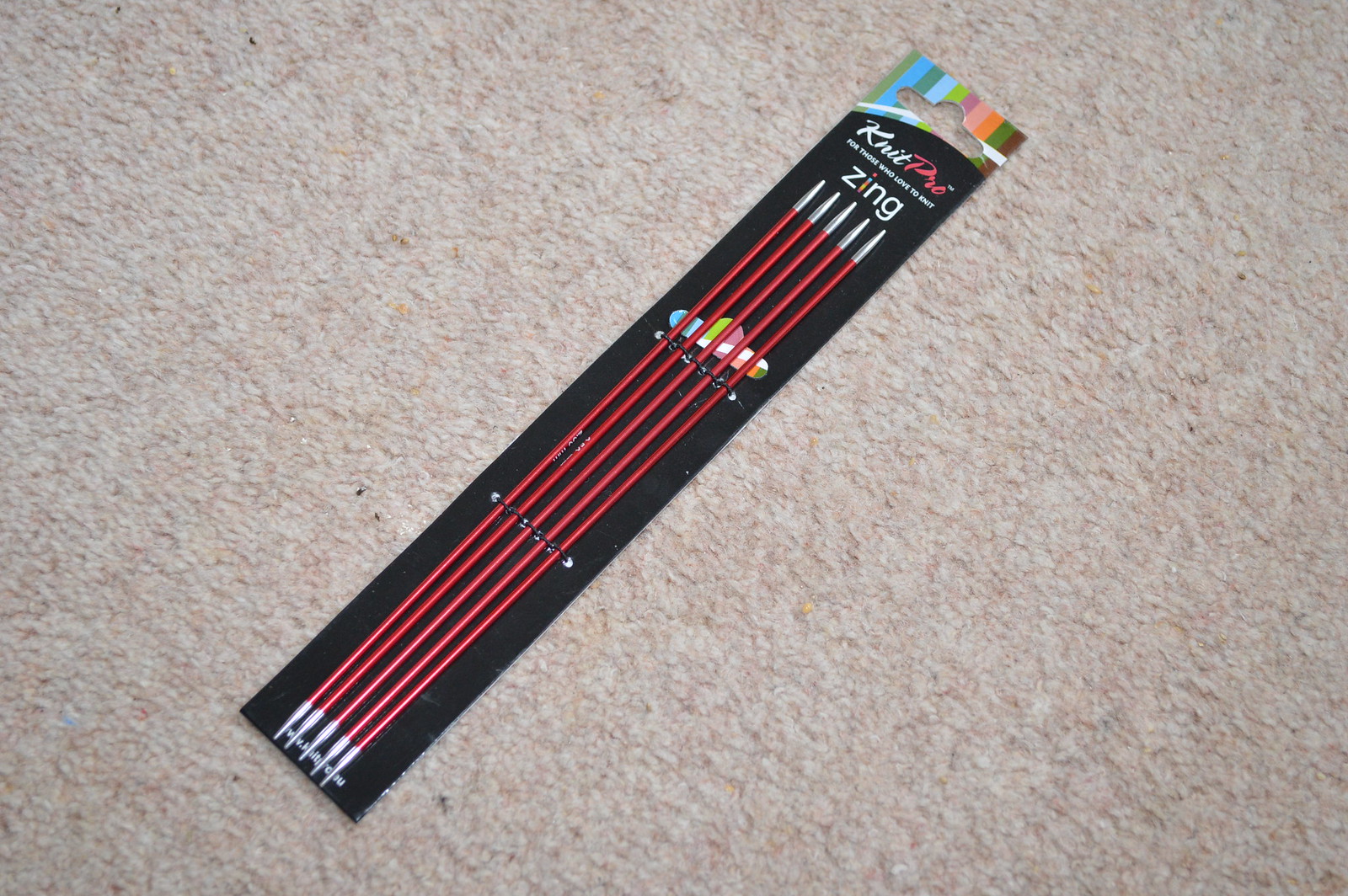The image depicts a color photograph of an unopened package of knitting needles resting diagonally from the upper right to the lower left on a beige, short nap carpet. The package has a thin, rectangular cardboard backing with a series of colorful stripes at the top in the following sequence: green, blue, green, blue, green, pink, orange, green, and brown. The brand name "Knit Pro" is prominently displayed in white letters, followed by the words "for those who love to knit" and "Zing" also in white. The packaging also includes a small hole for hanging on a display rack. The five knitting needles are made of red metal with silver tips on either end, and they are secured to the cardboard backing by two rows of thin black plastic strips.